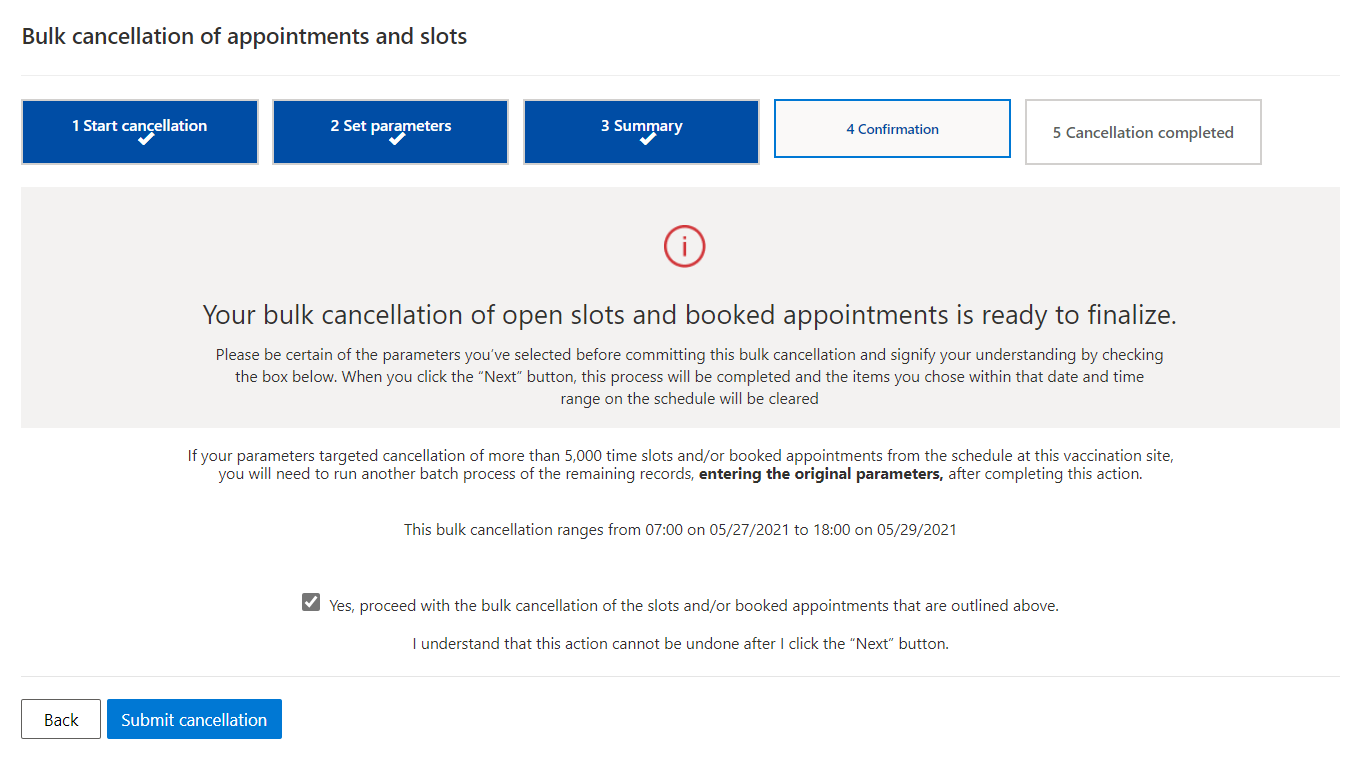"Volt Cancellation Process Overview

The image depicts a detailed interface for managing volt cancellation appointments and slots. The current progress is displayed across five steps, with the first three steps completed and highlighted in blue with checkmarks:

1. **Start Cancellation** - Blue button with a checkmark below.
2. **Set Parameters** - Blue box with a checkmark below.
3. **Summary** - Blue box with a checkmark below.

The process is currently on step four, which is indicated by a white box with "Confirmation" in blue text. Step five, "Cancellation Completed," remains unselected, marked by a white box with black text.

In the middle of the screen, a red circle with an 'i' icon alerts users with the message: "Your volt cancellation open slots and booked appointments are ready to finalize. Please be certain of the parameters you've selected before committing to this volt cancellation."

This section resides within a light gray box below the start cancellation steps. Additional information is provided about slot centers and booked appointments, including the total number of cancellations initialized, which exceeds 5,000. The detailed time range and date for the cancellations are also listed.

To proceed, users can check a box to confirm, and at the bottom left corner, a white "Back" button is available. On the right, a prominent blue "Submit Cancellation" button with white lettering allows users to finalize the cancellation."